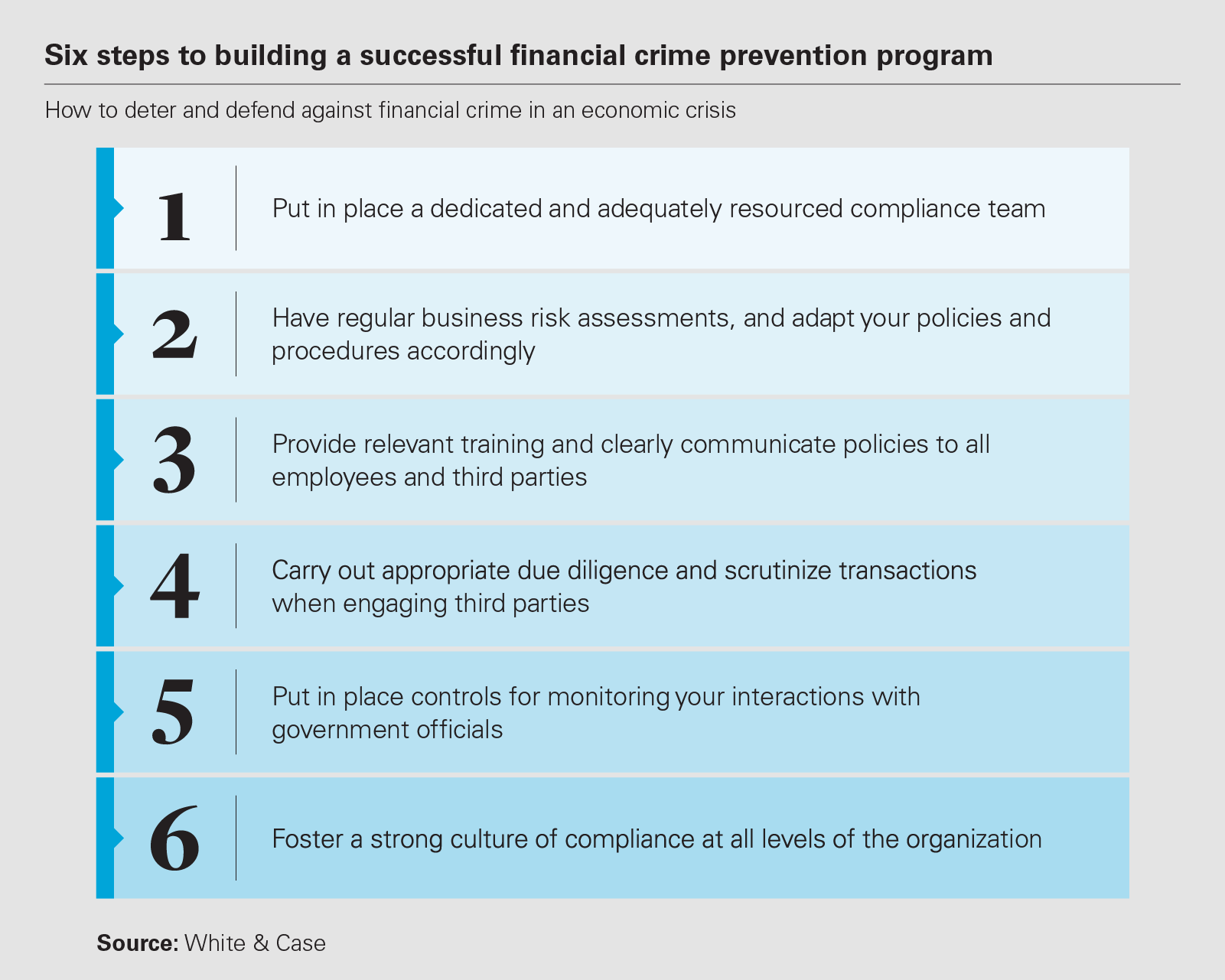The image is a square infographic with a light gray background, featuring a detailed six-step guide on building a successful financial crime prevention program. Across the top, bold black text reads "Six Steps to Building a Successful Financial Crime Prevention Program," followed by a thin horizontal rule and smaller black text stating, "How to deter and defend against financial crime in an economic crisis." Below this, there are six vertically stacked rectangles, each increasing in darkness from a light blue at the top to a darker blue at the bottom, forming a gradient. Each rectangle contains a step in the program, with bold serif numbers listed on the left. The steps are: 1. Put in place a dedicated and adequately resourced compliance team; 2. Have regular business risk assessments and adapt your policies and procedures accordingly; 3. Provide relevant training and clearly communicate policies to all employees and third parties; 4. Carry out appropriate due diligence and scrutinize transactions when engaging third parties; 5. Put in place controls for monitoring your interactions with government officials; and 6. Foster a strong culture of compliance at all levels of the organization. In the bottom left corner, the source is noted as "White & Case."